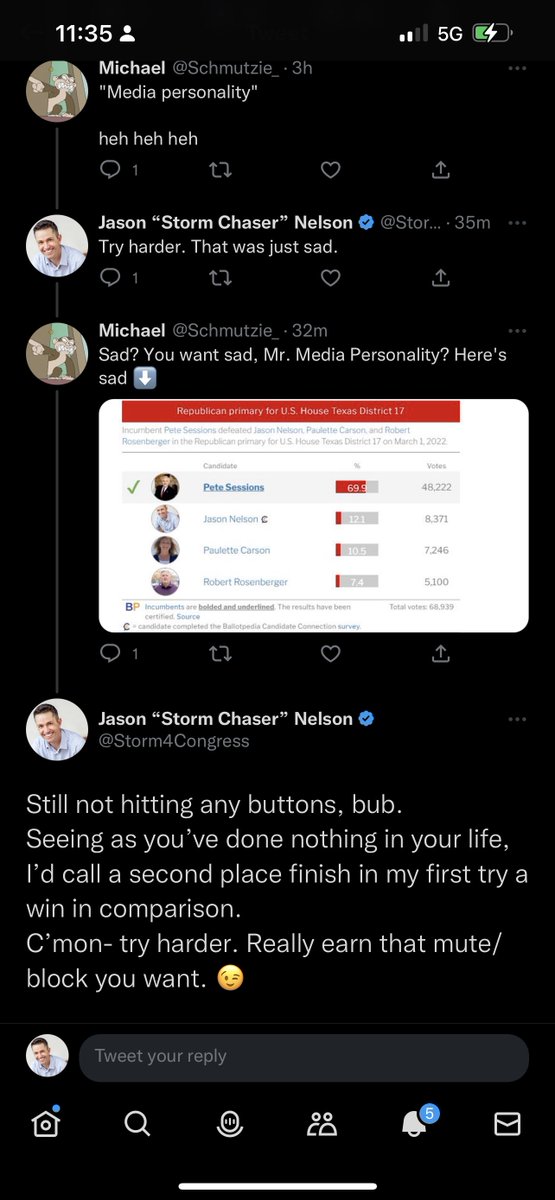The once notable time of 11:35 displays prominently on the screen. The signal strength is at 2 out of 4 bars, with 5G connectivity, and the battery level is at 50%. Michael is mentioned alongside a time span of 3 hours, and Dr. Nelson makes an appearance in the list of names. Among the contacts displayed are Paulette Carson, Robert Rosenberg, Jason Starcher, and Nelson. Despite no buttons being pressed, a sense of competition is implied, with a reference to achieving a second-place finish on a first attempt. A bold encouragement is given to win someone over and to let her earn them, with an optional use of a hash block.

The image sequence progresses, showing a person waking up, followed by a building depicted with a magnifying glass. A circle and underline emphasize specific details. A notification icon with a bell is visible, indicating five notifications. The final part of the sequence shows a person with a blank expression, and the background is entirely black.